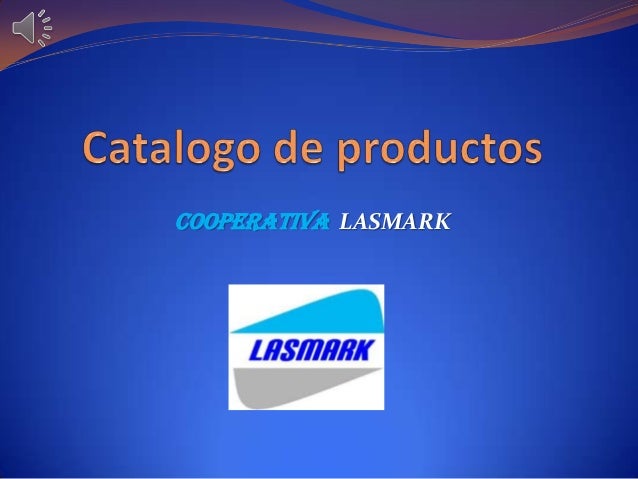The image features a product brand logo set against a gradient blue background that becomes brighter towards the center. At the top of the image, wavy lines in brown and purple blend seamlessly. The text at the center reads "Catalogo de Productos" in light brown or orange font, followed by "Cooperativa Las Marques" (alternatively noted as Cooperativa Lasmarc in some descriptions), where "Cooperativa" is in turquoise and "Las Marques" (or Lasmarc) in white. Toward the bottom of the image is a square logo on a white background. The dark blue, capitalized letters of "LASMARC" (or Las Marques) are centrally placed within the logo. Above the name, a light blue upward-sloping hill contrasts with an inverted gray hill below. Additionally, a lit speaker icon with speckles is positioned in the top left corner, indicating active audio.